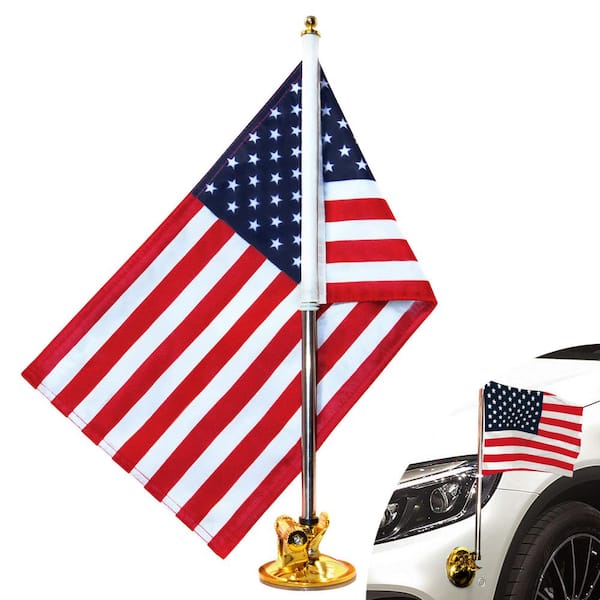This photograph captures an American flag prominently displayed, showcasing its iconic red and white stripes alongside a blue field adorned with white stars. The flag is fixed to a short silver pole, topped with a gold finial, and secured to a gold base. The pole is mounted on the front of a white vehicle, positioned just below the headlight. The vehicle's front quarter, including the tire, fender, and headlight, is visible. Additionally, there is a semi-circular inset photo in the bottom right corner of the image, highlighting the flag and its mounting on the vehicle. The overall composition draws attention to the patriotically decorated car front.